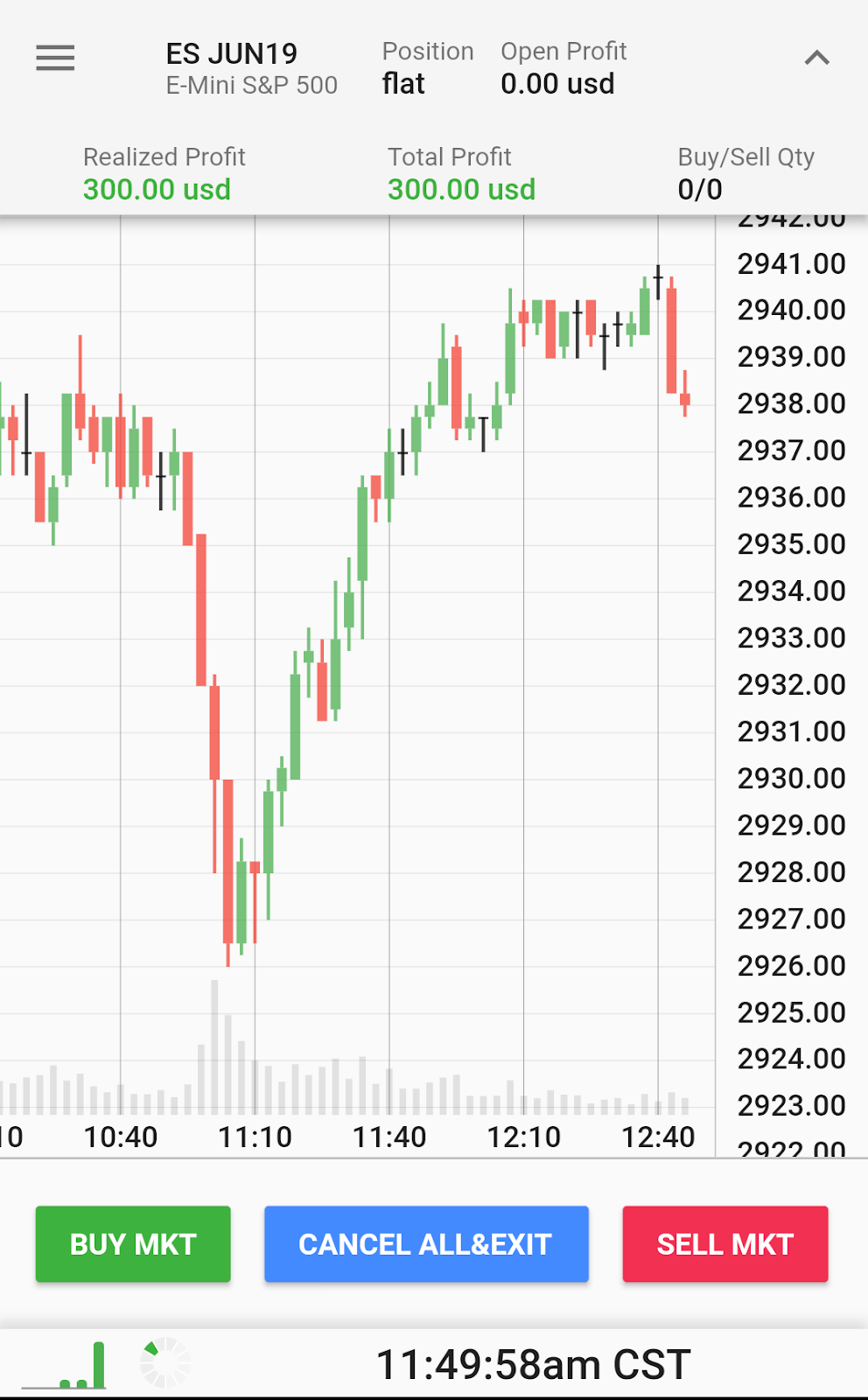The image portrays a detailed stock market projection for June 19th, set against a light gray background. 

In the upper left corner, three vertically stacked lines can be seen. Adjacent to these lines is black text that reads "ES June 19." Below this, in smaller black font, it says "E Mini S&P 500."

The next section down is labeled "Position," followed by the word "Flat." Below this, "Open Profit" is indicated, with a subsequent figure of "0.00 USD."

On the far right side of the image is an upward-pointing directional arrow. Beneath this arrow is a series of labels and corresponding values:
1. "Realized Profit" is displayed in black text, followed by a green figure showing "$300 US."
2. "Total Profit" is also shown in green text, with the same amount, "$300 US."

To the far right, there are labels for "Buy," "Sell," and "Quantity," with each showing a value of "0.00" beneath them.

Below these text elements, a graph illustrates the market's fluctuation, ranging from around 29.37 up to 29.40 and down to 29.24. The time intervals marked on the graph span from 10:40 to 12:40.

Underneath the graph is a legend, including three color-coded rectangles. A green rectangle with white text reads "Buy Market," a blue rectangle with white text says "Cancel All and Exit," and a red rectangle with white text indicates "Sell Market."

At the bottom of the image, the current time is displayed in black text as "11:49 and 58 seconds AM CST."